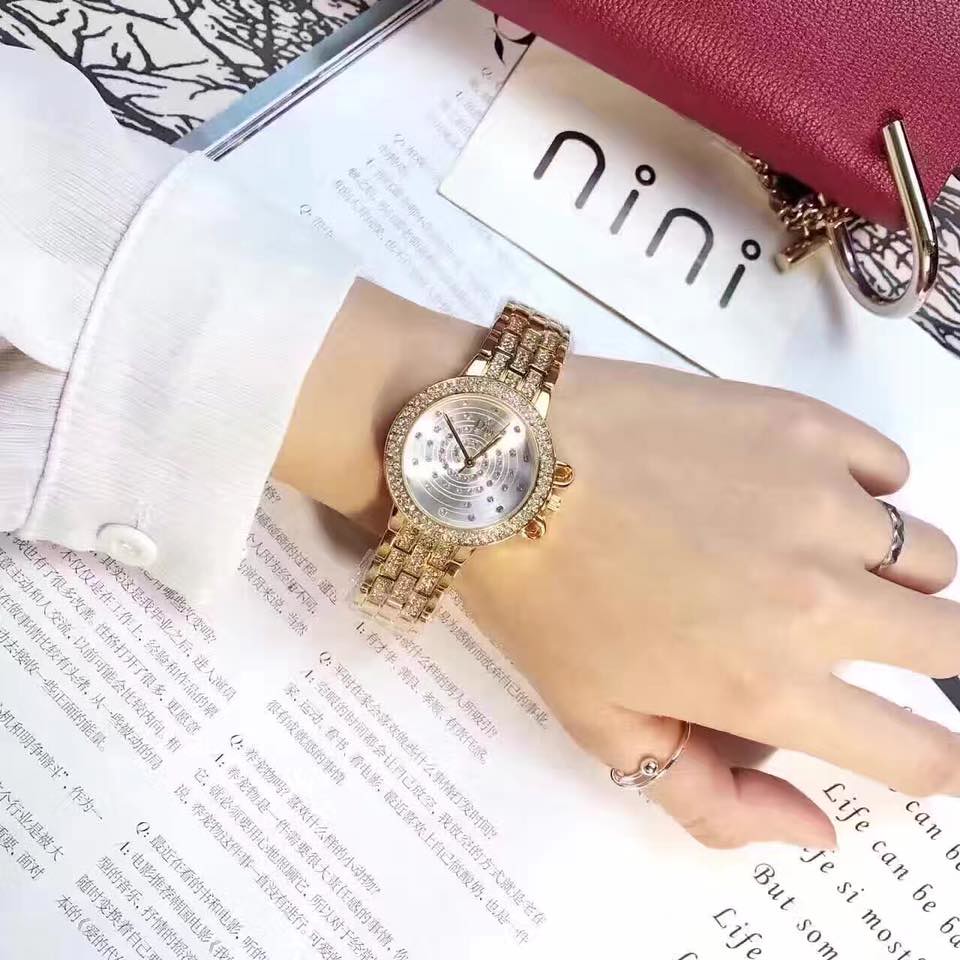The image features a woman's left hand adorned with an extremely ornate and luxurious watch. The watch has a golden band embedded with diamonds around its rounded edges and face, which also showcases diamond-like dots. The watch's hands point to 11 and 1, and the face includes platinum or silver decorations. The woman is wearing a white long-sleeve button shirt and has rings on her thumb and ring finger, which are more silver in color.

The hand appears to be resting on two pieces of white paper. One of these papers, situated below the wrist and covering most of the bottom half of the hand, is filled with dense Asian characters. The other paper, located below the fingers, contains English words that include "can," "life can be," and some French text like "see most."

Above the wrist is another piece of white paper, which reads "nini" in large text with little circles instead of dots above the "i"s. Above this paper, towards the top of the image, is a red or burgundy bag with a silver clasp around the nearest corner and edge.